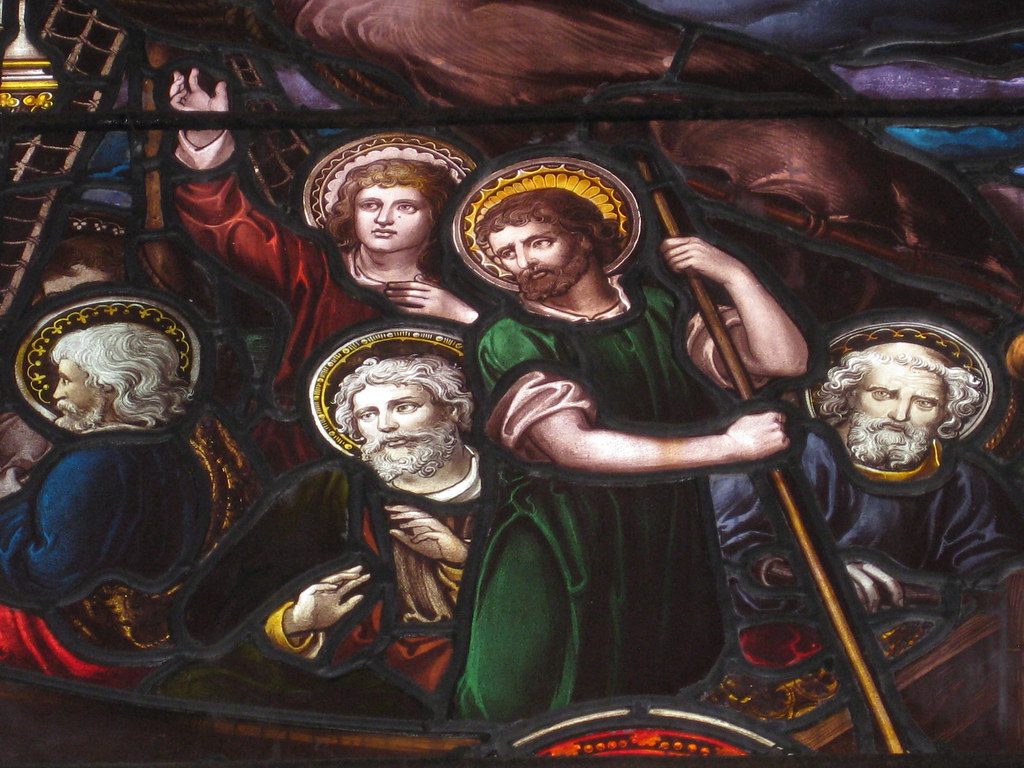This image features an intricately detailed stained glass window memorial in St. Kilda Presbyterian Church, St. Kilda, South Melbourne, Victoria, Australia. It depicts the biblical scene of Jesus calming the storm with His disciples in their boat. Jesus, distinguished by a green robe and a cylindrical halo painted around His head, stands prominently in the foreground holding a long staff that extends to the right. Surrounding Him are His disciples, each adorned with cylindrical halo shields. They have deeply detailed facial features and gray wavy hair, with their flowy robes in shades of blue, green, and red. Notably, one individual in the back, possibly with an effeminate appearance, raises a hand towards the upper left. The disciples, also dressed in intricate robes, display expressions of concern and awe, particularly the older man in a blue robe and another young man in red. The composition captures a dynamic moment of divine intervention amid a storm, reflected through the movement and postures of the figures, evoking a sense of spiritual reverence and historical artistry.